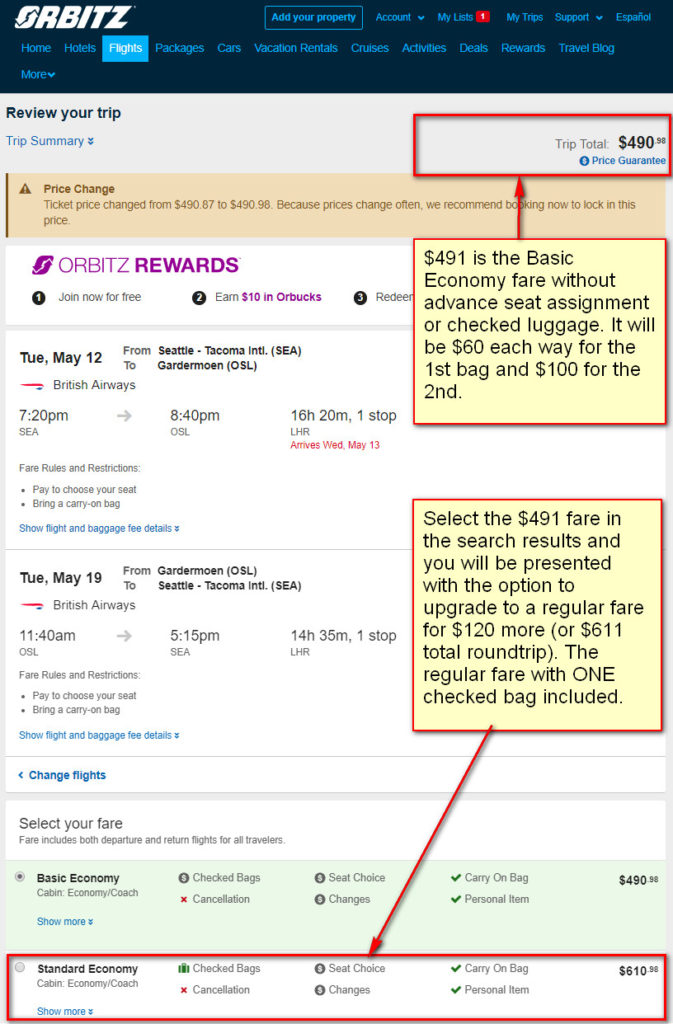This detailed screenshot captures various elements of a travel booking website interface:

At the top of the page, a dark blue banner spans approximately 10% of the screen's height. On the left side of this banner, the white Orbits logo is prominently displayed in all capital letters. Adjacent to the logo, the navigation menus are highlighted in teal text. 

The first item, "Add your property," appears enclosed in an outlined button. To its right is "Account" with a drop-down arrow, followed by "My Lists" which includes a small red box displaying an unreadable number, presumably a counter. Continuing to the right, the menu lists options such as "My Trips," "Support" (with a drop-down arrow), and "Español" for language settings.

Directly beneath the top banner is the main navigation menu, beginning with "Home," "Hotels," and "Flights." The "Flights" option is highlighted with a teal background and white text, indicating it is currently selected. Additional menu items include "Packages," "Cars," "Vacation Rentals," "Cruises," "Activities," "Deals," "Travel Blog," and lastly, "More" with a drop-down arrow.

The main content section, set against a white background, starts with "Review Your Trip" in the upper left. Below it, the section labeled "Trip Summary" is in light blue with two down arrows. On the right side of this area, the "Trip Total" is displayed as $490, with "Price Guarantee" written in blue beneath it, accompanied by a small blue information icon.

A notable feature is the overlaid red rectangle surrounding the "Trip Total" and "Price Guarantee," drawing attention to this area. Further detailed explanations are provided in subsequent outlined sections below this highlight.